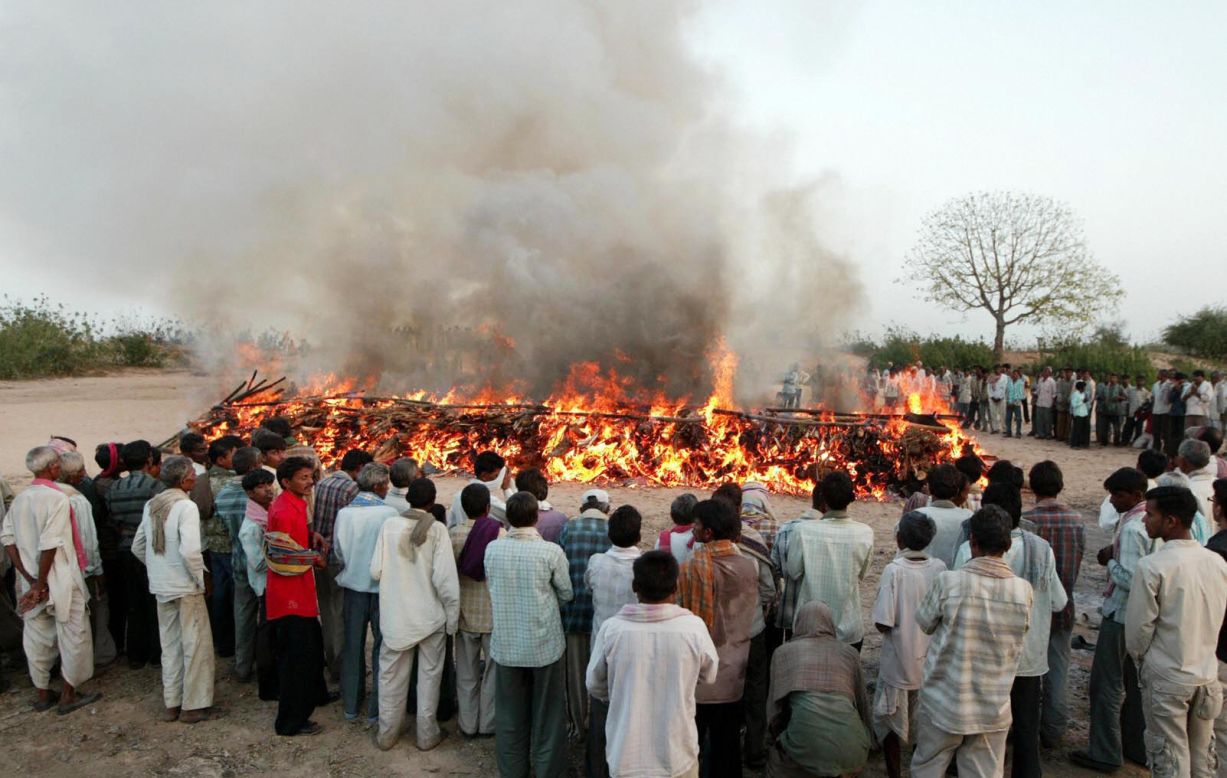The image depicts a horizontal rectangular scene capturing a large fire in what appears to be an organized setting. The fire, contained within a rectangular area, is spreading wide but has not yet reached its full intensity, emitting mostly dark gray smoke that lightens as it ascends into the overcast, gray sky. Surrounding the fire is a dense crowd of people, predominantly men, standing several rows deep, all with their backs to the camera and focused intently on the flames. The men, who appear to be of African or Kenyan nationality, are dressed primarily in pants and shirts, many wearing scarves around their necks. The fire itself consists of a variety of materials, including sticks and possible brush, although no logs are visible. There is no firefighting equipment in sight, and the background reveals some buildings beyond the crowd. Further up on the right side, additional onlookers can be seen observing the scene. The overall atmosphere suggests a deliberate and organized gathering in an outdoor setting.